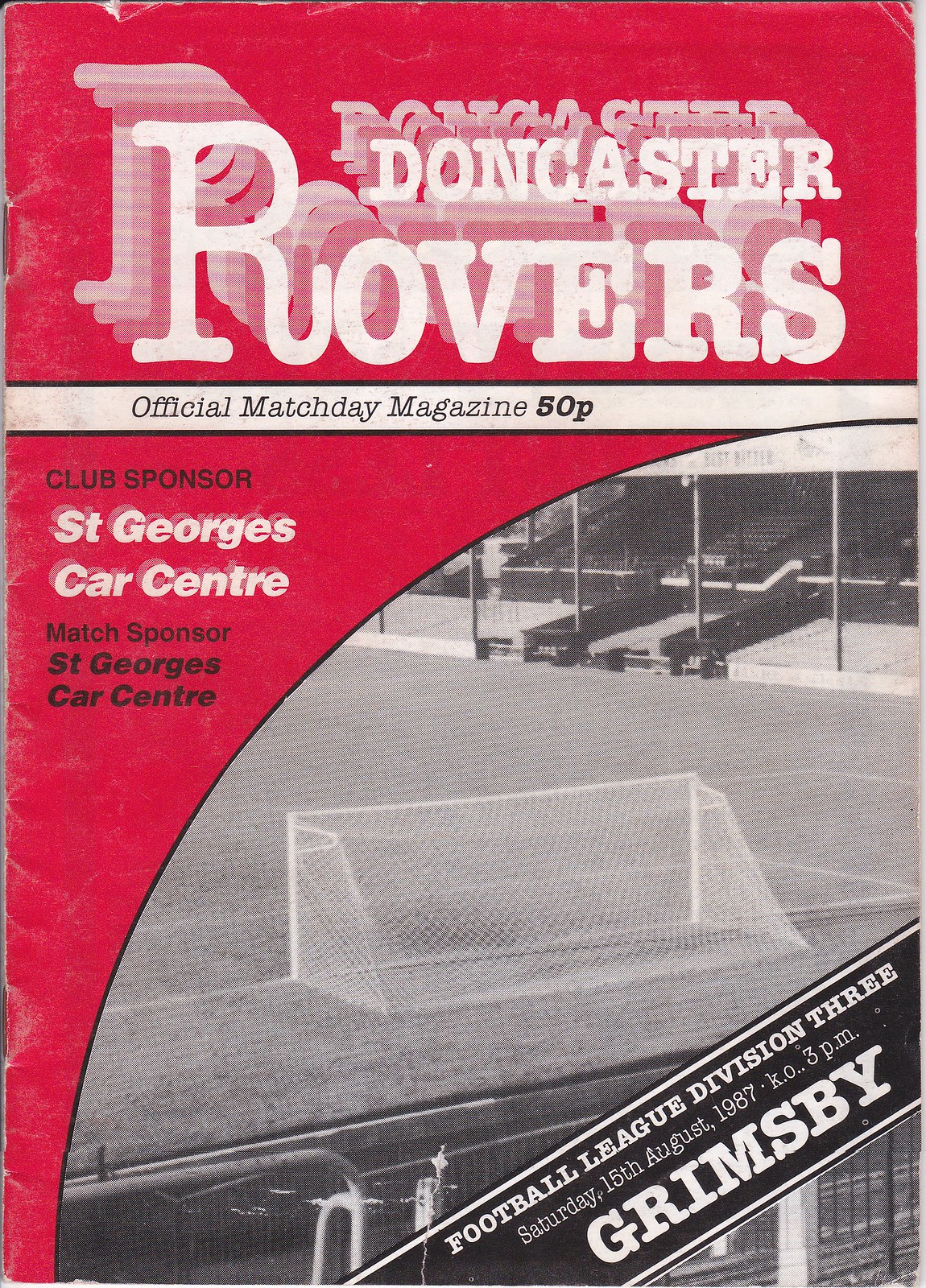This image is a red background front cover of an old, weathered soccer program for the Doncaster Rovers, dating back to Saturday, 15 August 1987. At the very top, "Doncaster Rovers" is prominently displayed in white letters. Just below, a thin white strip reads "Official Match Day Magazine 50P." The club and match sponsor, St. George's Car Centre, is mentioned twice in the red background area beneath this strip. On the right-hand side, there's a grainy, black and white oval photograph depicting a football field with a goal post and spectator stands. A diagonal black strip with a white border cuts across the bottom right corner, displaying essential match details in white font: "Football League Division III, Saturday 15 August 1987, KO 3 PM," followed by "Grimsby" in large capital letters.